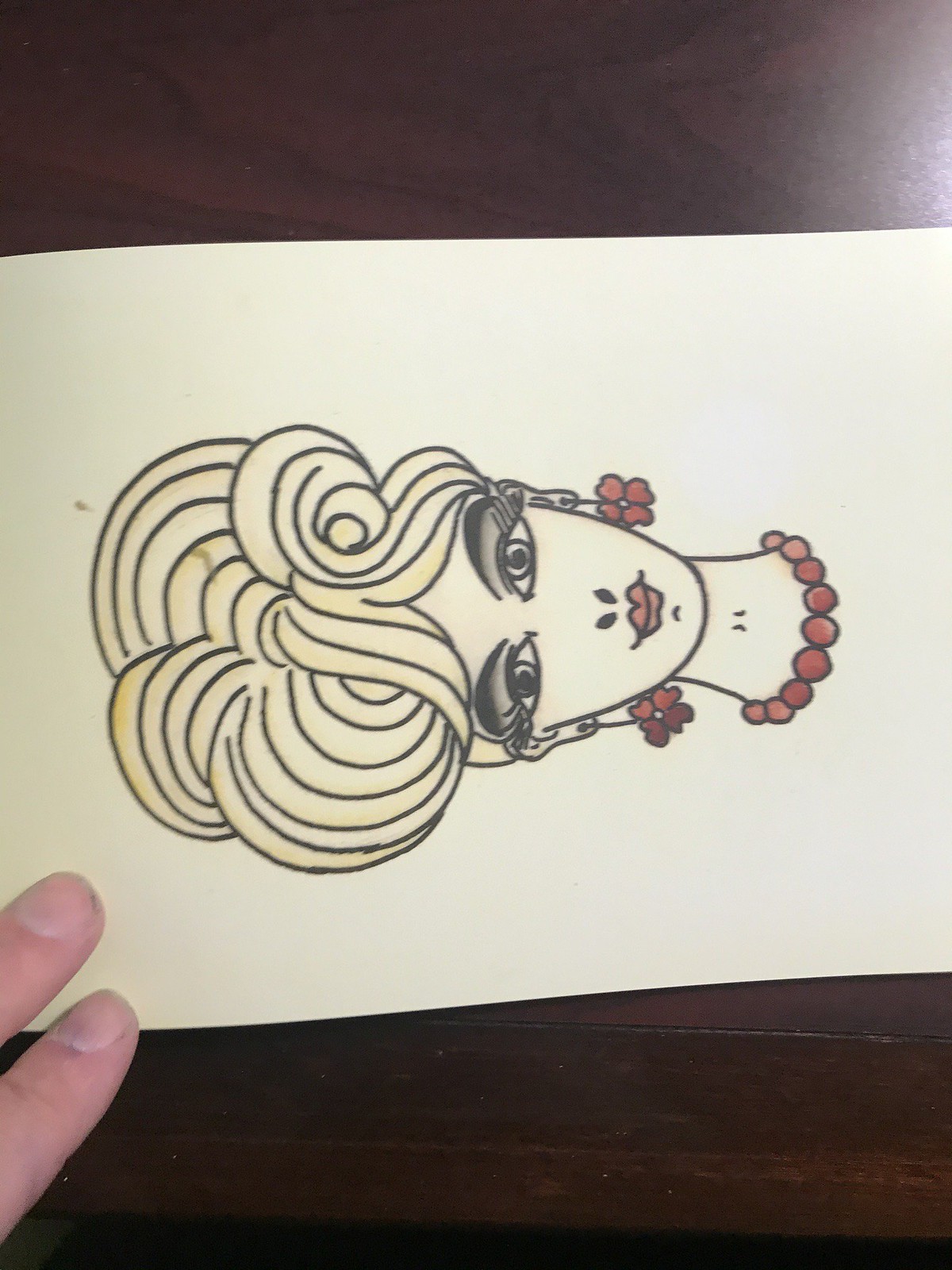The image depicts a detailed colored pencil drawing of a young woman with an oval-shaped face, held down at the top left corner by two human fingers against a wooden board. The drawing is oriented vertically, set on an eggshell white paper with a black background. The woman features striking yellow hair styled in an elaborate wavy updo, which sits atop dark, thick eyebrows, and almond-shaped, wide eyes enhanced by heavy makeup and long eyelashes. She has a small nose, red rosebud lips, and is adorned with dangling, flower-shaped earrings and a matching red beaded necklace. The round red beads and earrings add an elegant touch to her slim neckline.